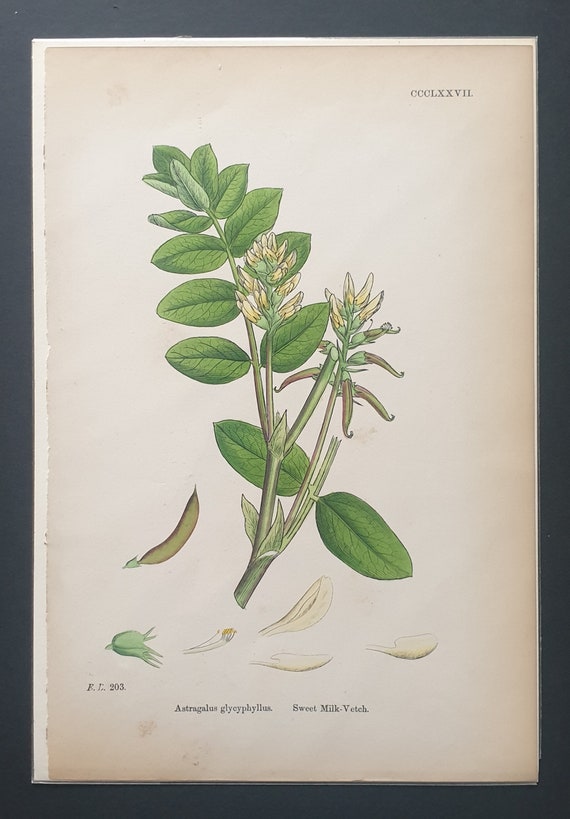A vertically rectangular, framed print of a botanical drawing, set against a light brown, aged vellum-like background with a thin white border. The frame is black. At the top right of the illustration are the Roman numerals CCCLXXVII in black letters. The centerpiece is an artistic yet scientifically detailed depiction of a plant known as Astragalus glycyphyllos, or Sweet Milk Vetch. The plant features a main stem with branches extending out, bearing small oval-shaped green leaves with a distinct center vein and finer veins radiating from it. Two stalks with yellowish flower buds emerge from the branches, not yet in full bloom. Below the main illustration is some black text: "FT203." and the plant's scientific name, "Astragalus glycyphyllos," followed by its common name, "Sweet Milk Vetch."